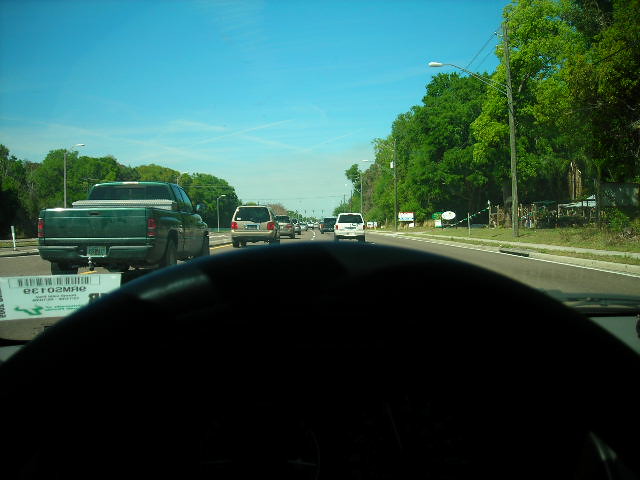The photograph captures a driver's view from inside a car, with the black semi-circle of the steering wheel dominating the bottom half of the image. Positioned at the lower left corner of the windshield is an emissions inspection sticker featuring a black UPC code and some unreadable details, with a green strip at the bottom. Through the clear window, a bustling two-lane road extends ahead under a light blue sky dotted with white clouds. Directly in front of the car, a white SUV leads the way with a dark green pickup truck and a gold or bronze SUV visible in the left lane. Further ahead, more vehicles are discernible along with traffic lights in the distance. On the far right, there is a curb lined with grass, and a building partially obscured by a row of trees. Streetlights and overhead wires stretch out against the backdrop of greenery, revealing it to be a sunny day.